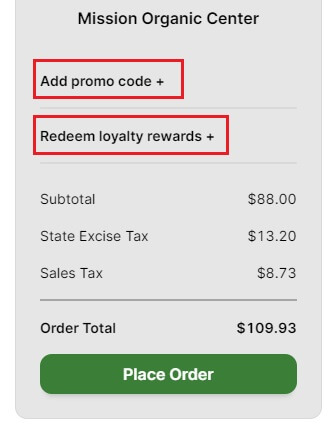This is a screenshot snippet of a checkout section from Mission Organic Center. The layout features a light gray background with various elements organized for clarity. At the top, centered in black text, is the name "Mission Organic Center."

Immediately below the title, there are two highlighted sections bordered in red rectangles. The first red rectangle is left-aligned and contains the text "Add Promo Code" and a plus symbol. Separating this section is a thin light gray dividing line.

The next highlighted section, also bordered by a red rectangle, contains the text "Redeem Loyalty Rewards" accompanied by another plus symbol. Beneath this is another thin gray dividing line.

Below these options is a table detailing the monetary breakdown of the order. The table has two columns: the left column lists the entries "Subtotal," "State Excise Tax," and "Sales Tax." The corresponding amounts are right-aligned in the right column as "$88.00," "$13.20," and "$8.73," respectively.

A darker gray dividing line separates the table from the order summary. The text "Order Total" is displayed, followed by the total amount right-aligned as "$109.93."

At the bottom of the box, there is a green action button containing the white text "Place Order."